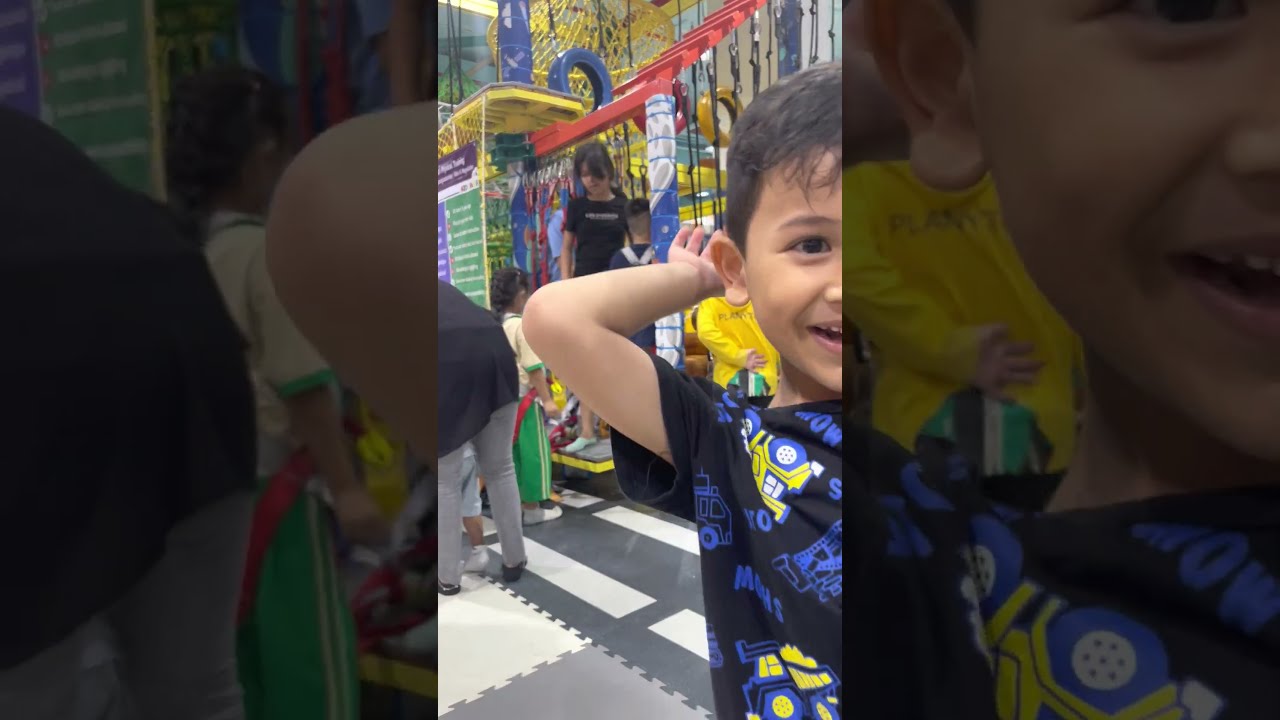In this vibrant image of an indoor playground, the central figure is a young boy, half of his body visible, grinning widely with excitement. He's wearing a black t-shirt with blue and yellow designs, possibly of construction trucks. The boy’s arm is bent at the elbow, with his hand positioned behind his head. The scene around him is bustling with activity: on his left, a small girl dressed in a yellow shirt, green pants, and white shoes stands out. Behind them, an older woman is bent over, attending to a toddler, who remains mostly out of sight with only their legs visible between the woman's. The background reveals a colorful playground with varied structures, such as ropes, steps, and slides in bright hues of yellow, red, blue, and green. Amidst the lively setting, a young girl acts as the gatekeeper in a caged-in play area, managing the children's entrance as space becomes available, adding to the joyful confusion typical of a children's amusement space.